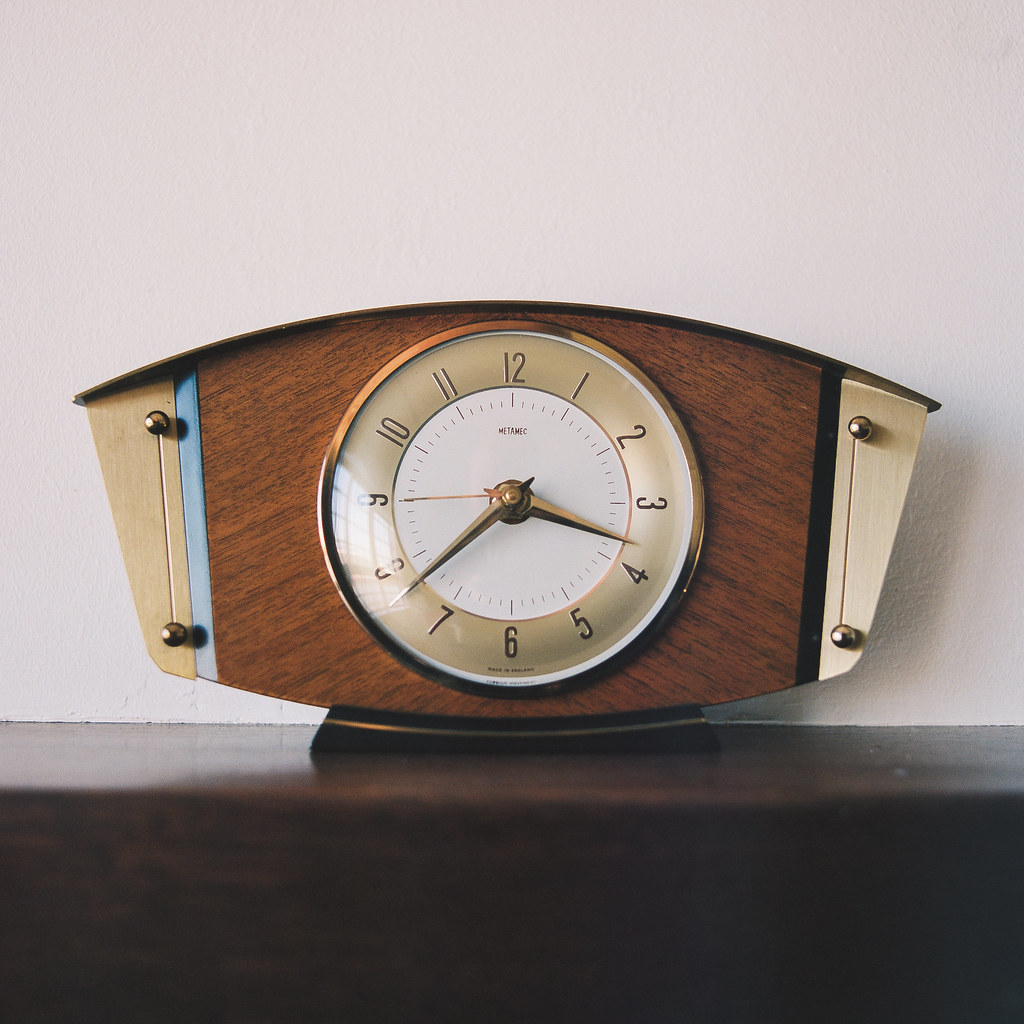The image features an intriguing analog clock positioned centrally on a dark-stained wooden table, set against a whitish gray wall. The clock's design blends modern and traditional aesthetics, housed in a geometric frame that isn't quite rectangular nor oval, but showcases a rich walnut woodgrain. The top and bottom edges of the clock frame curve slightly downward and upward respectively, contributing to its unique shape. 

The clock face itself is situated in the center of the wooden frame, ringed by a tan or beige outer rim and a white inner circle. Black numbers, indicating hours 1 through 12, are placed on this tan or gold-colored background. Markings for the seconds encircle the central point where the hands pivot, resting against the white backdrop. The hour and minute hands are in a gold or brass hue, with a striking red second hand adding a touch of contrast.

Flanking the clock on either side, two brass knobs linked by vertical strings add to the distinctive design. Small screws are visible, hinting at the functionality embedded in its form. While the exact brand of the clock is too diminutive to discern, the overall composition and materials convey a blend of modern craftsmanship with timeless elements.